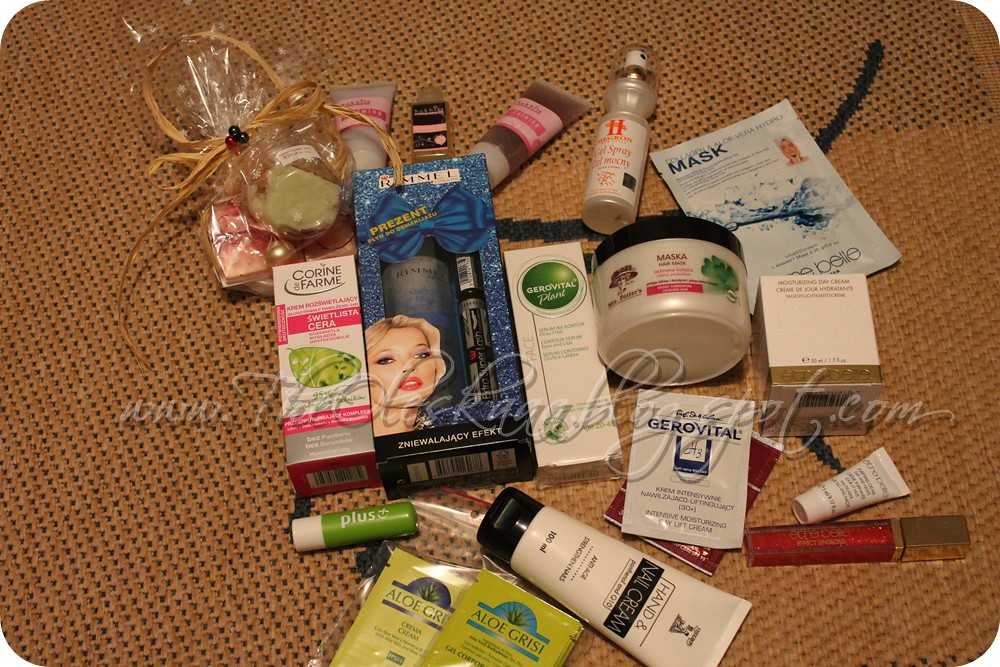A diverse collection of cosmetic products is arranged on what appears to be a woven mat or an orange carpet with black dots, though it's unclear if these dots are actually openings. The image is partly obscured by a script-font watermark that reads "www.thesomethingblogspot.com," though the lightness of the watermark and the texture below make it difficult to decipher.

In the foreground, there is a cellophane-wrapped bundle tied with a sisal ribbon adorned with three small berries. The contents of the bundle are not visible. Attached to it are several cosmetic items: a white squeeze tube with a pink label, a small bottle with a black label featuring pink writing, and another squeeze tube similar to the first but containing a brown or deep purple substance.

Adjacent to the bundle is a tall, slender spritz bottle labeled as a gel spray, with a logo resembling two pillars crossed to form an "H." There is also a sealed envelope labeled "Aloe Vera Hydro Mask."

In the next row, there are various boxes and containers: 
1. A box labeled “Chlorine and Pharma Sweet Listacera,” notable for its white and pink packaging and a picture of something green.
2. A blue box, larger in size, which seems to contain mascara and a bottle, adorned with a blue bow. The text on the box appears to be in a non-English language, possibly Polish.
3. A white box with green lettering labeled "Giro Vital Plant."
4. A squat, wide jar with a black top containing a tan or silvery substance, labeled “Nazca.”

Further items include:
- A cubicle box labeled as "Moisturizing Skin Cream."
- A lip balm with a prominent "+" sign.
- A squeeze tube of hand and nail cream.
- Another product from Giro Vital: an "Intensive Moisturizing Lift Cream."
- Lastly, there are a couple of packets resembling tea bags labeled "Aloe Greasy Crema."

This image showcases a diverse array of skincare and cosmetic products, indicative of a well-curated collection aimed at various aspects of personal care and beauty routines.